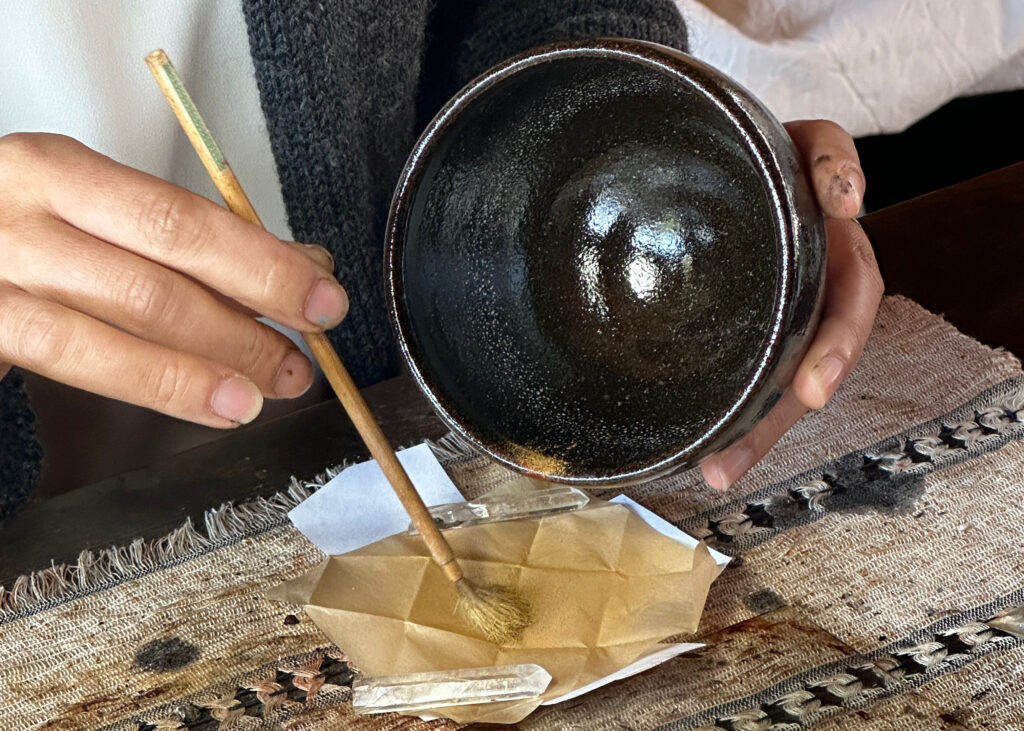In this detailed photograph, the focus is on a pair of hands engaged in an intricate art process. The painter is delicately balancing a shiny, slate gray ceramic pot in one hand and a light brown, fluffy-bristled brush in the other. This pot, possibly coated with a reflective glaze, contains a mysterious brownish-yellow powder. The artist is seen pouring the powder onto a tan piece of paper, which is meticulously folded to form a square pattern. The paper rests on a table covered by an old, frayed, and striped cloth—speckled with stains from previous artistic endeavors, likely from paint or dyes. The painter's white and gray sweater adds a subtle contrast to the scene, with their dirty fingernails hinting at the hands-on nature of their craft. The interplay of materials and textures, from the ceramic pot to the folded paper and the stained cloth, captures the essence of an artist deeply immersed in their creative process.